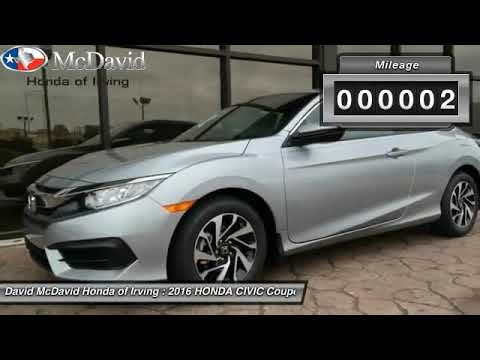The advertisement features a sleek, silver 2016 Honda Civic Coupe prominently in the center, positioned slightly facing to the left. The car is distinguished by its black tires with silver rims, exuding a sporty appeal. The backdrop showcases the reflective glass exterior of a building, adding a modern touch to the scene.

In the upper left-hand corner, an oval logo adorned with the Texas flag and an overlay of a silver Texas silhouette captures attention. Adjacent to this emblem, 'McDavid' is elegantly inscribed in silver lettering, with 'Honda of Irving' written in black font just below it.

On the top right corner, a rectangular box features the word 'Mileage' and beneath it, in a black square, the car’s mileage is displayed as '000002', suggesting the vehicle is practically brand new.

Finally, along the bottom edge of the advertisement, a gray banner stretches horizontally, presenting the dealership’s name and car details: 'David McDavid Honda of Irving, 2016 Honda Civic Coupe'.